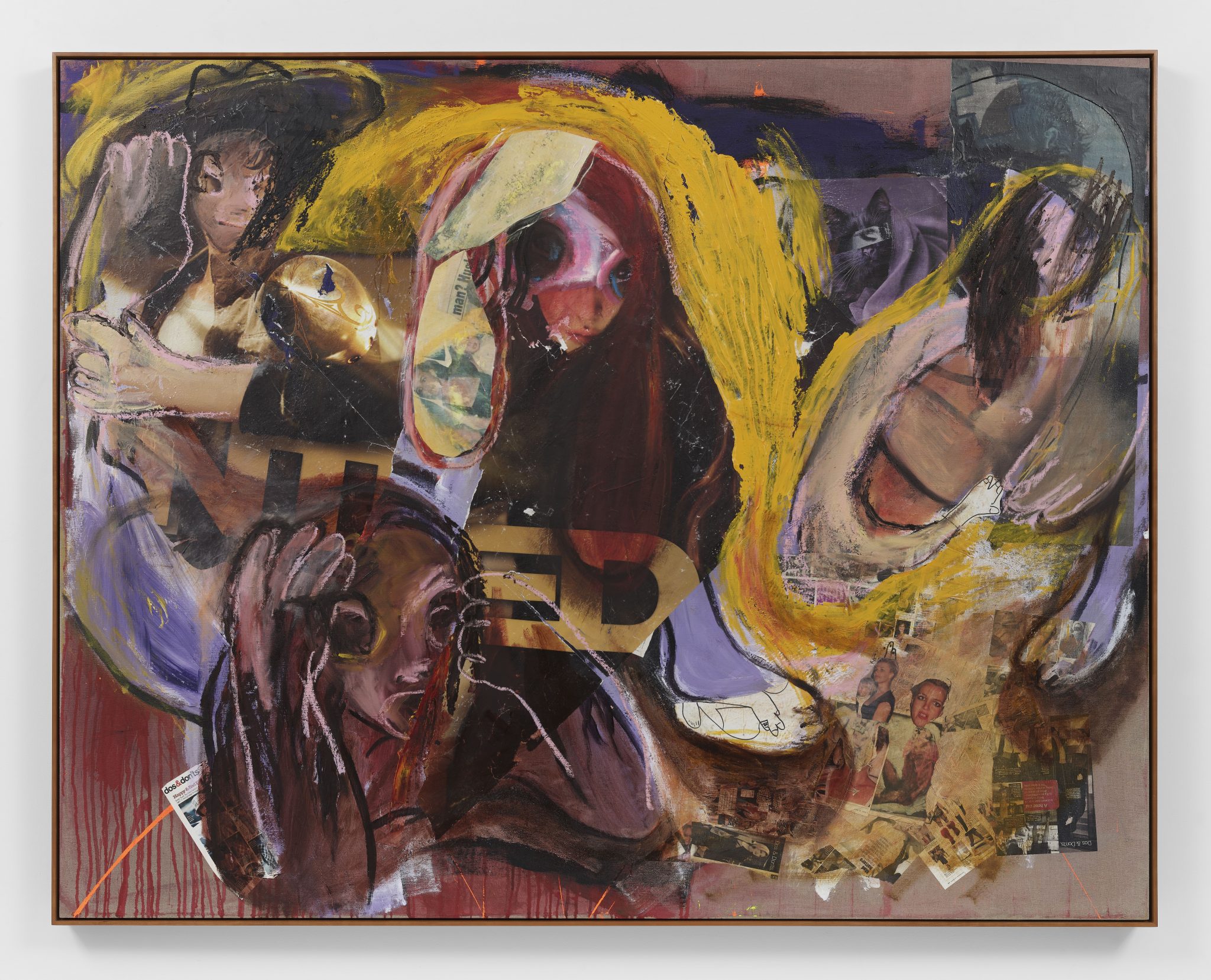The image depicts a layered and complex Impressionist artwork, framed in white. This partially abstract painting is a collage of caricatured and realistic human figures. Dominantly, there are several prominent, vividly detailed faces that stand out. On the upper left, a character wearing a large hat and a vertical black and white striped shirt is noticeable, though the gender is indistinguishable. Near this figure, there appears to be a person in a mask and cowl, with a brass belt and a pouch. In the center of the painting, a figure with red hair and a possible headdress has a bruised face, suggesting themes of abuse.

In the bottom left corner, there is a striking figure of a woman, with hands on her head, seemingly in a state of despair. Echoing this sense of distress, another person resembling a 'tin man' has gloves on, shielding their eyes from an invisible horror. The lower right corner of the artwork showcases photographic clippings of real-life women's faces, likely extracted from fashion ads, advertisements, or gossip magazines. These juxtaposed images within the artwork might be hinting at societal issues or critiques, adding a haunting realism to the abstract sketch-like quality of the painting. The painting combines elements of Impressionism with abstract caricatures, invoking an emotional, reflective response through its detailed eclectic elements.